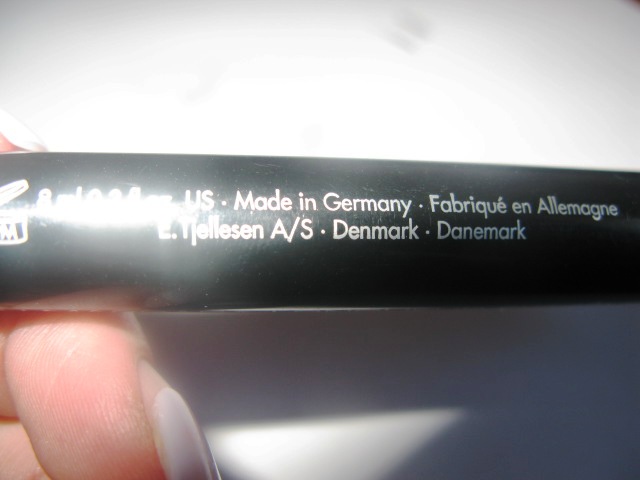This image features a close-up of a black pen with a white background. The pen's glossy finish partially obscures the text due to a camera flash, creating a glare primarily on the left side of the pen. Despite the glare, the visible white text on the pen reads: "Made in Germany, Fabrique in Allemagne, Denmark, Denmark." The pen is held by a woman whose index finger, adorned with white fingernail polish, is visible in the lower left corner of the image. The lighting creates distinct shadows beneath the pen, which adds depth to the otherwise all-white background.